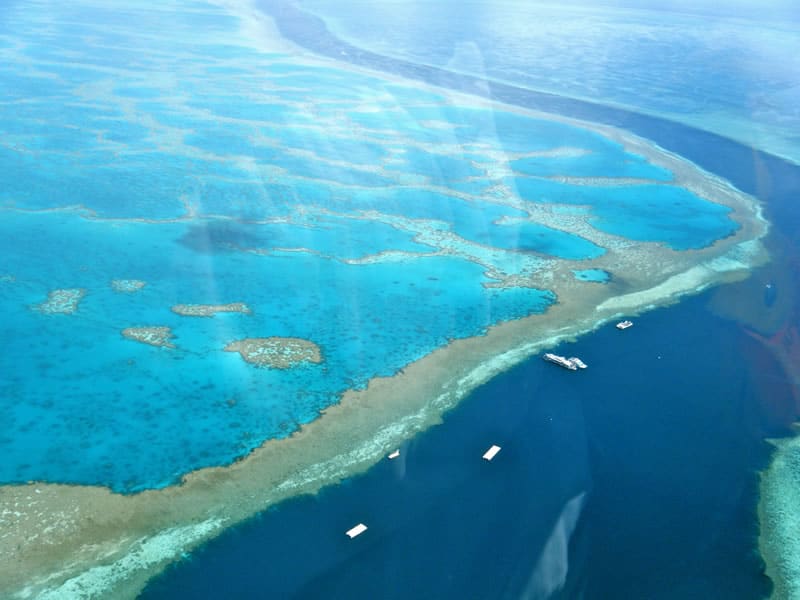This horizontal rectangular, color image presents an aerial or bird's-eye view, likely taken through an airplane window, as evidenced by the faint reflection of the glass. The scene captures a striking contrast between deep blue and lighter aquatic hues. At the center, a deep blue river snakes its way from the bottom right, curving up and slightly left, before narrowing and heading towards the top left quadrant of the frame. This river is flanked on either side by tan sandy banks, giving way to a lighter aqua-blue expanse, reminiscent of a coral reef or large natural aquatic formation. Scattered within the dark blue channel are several small white boats, appearing as tiny white rectangles, enhancing the image’s sense of scale. Adjacent to the river on the left side, a narrow light brown beach subtly separates the flowing waters from the surrounding lighter blue pools, completing a vivid depiction of this coastal or riverine landscape.